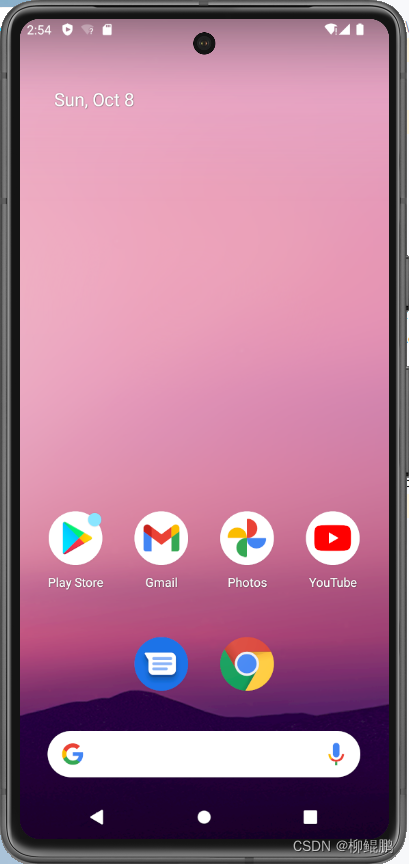The screenshot features a cell phone display with a gradient background starting from light purple at the top and transitioning to a darker purple about two-thirds of the way down, eventually blending into a dark blue or black mountain silhouette. 

At the very top of the screen, the time "2:54" is displayed in white font, alongside icons for battery life and phone signal strength on the top-right corner. The top-left corner shows the strength of the internet connection.

A few inches below, in gray letters, it reads "SUN, OCT 8," indicating the day, month, and date. Below this date information, several app icons are arranged in a grid-like pattern:

1. **Play Store** - A white circle containing a multi-colored play button in blue, green, yellow, and red.
2. **Gmail** - A white circle featuring a large "M" in red, yellow, blue, and green.
3. **Photos** - A white circle with a multi-colored pinwheel-like icon.
4. **YouTube** - A white circle with a red rectangle and a white play triangle in the center.
5. **Texting App** - A blue button with a piece of paper displaying lines, symbolizing text messages.
6. **Google Search** - An icon with the typical Google colors: green, blue, red, and yellow. 

These apps are displayed prominently against the phone's colorful background, providing quick access to essential functions.